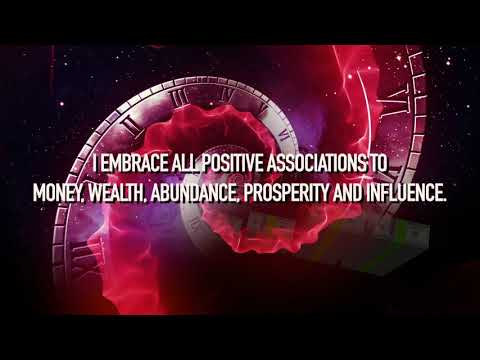The image features a central graphic of a twisted, spiral-shaped clock adorned with Roman numerals, set against a stunning space-themed background. The clock appears fragmented and contorted, creating a dynamic, swirling pattern that reaches both the upper right and left sides. This spiral is accompanied by flowing, reddish streaks that resemble a twisting scarf, adding an abstract, ethereal quality. The background is a deep black, peppered with white stars and hints of a purple galaxy, enhancing the cosmic atmosphere. Large black bars frame the top and bottom of the image, reminiscent of widescreen borders. Dominating the center of the image, in bold white capital letters with a drop shadow effect, is the motivational text: "I embrace all positive associations to money, wealth, abundance, prosperity, and influence." A faint, nearly imperceptible watermark can be seen, suggesting the creator's signature is subtly embedded in the design.